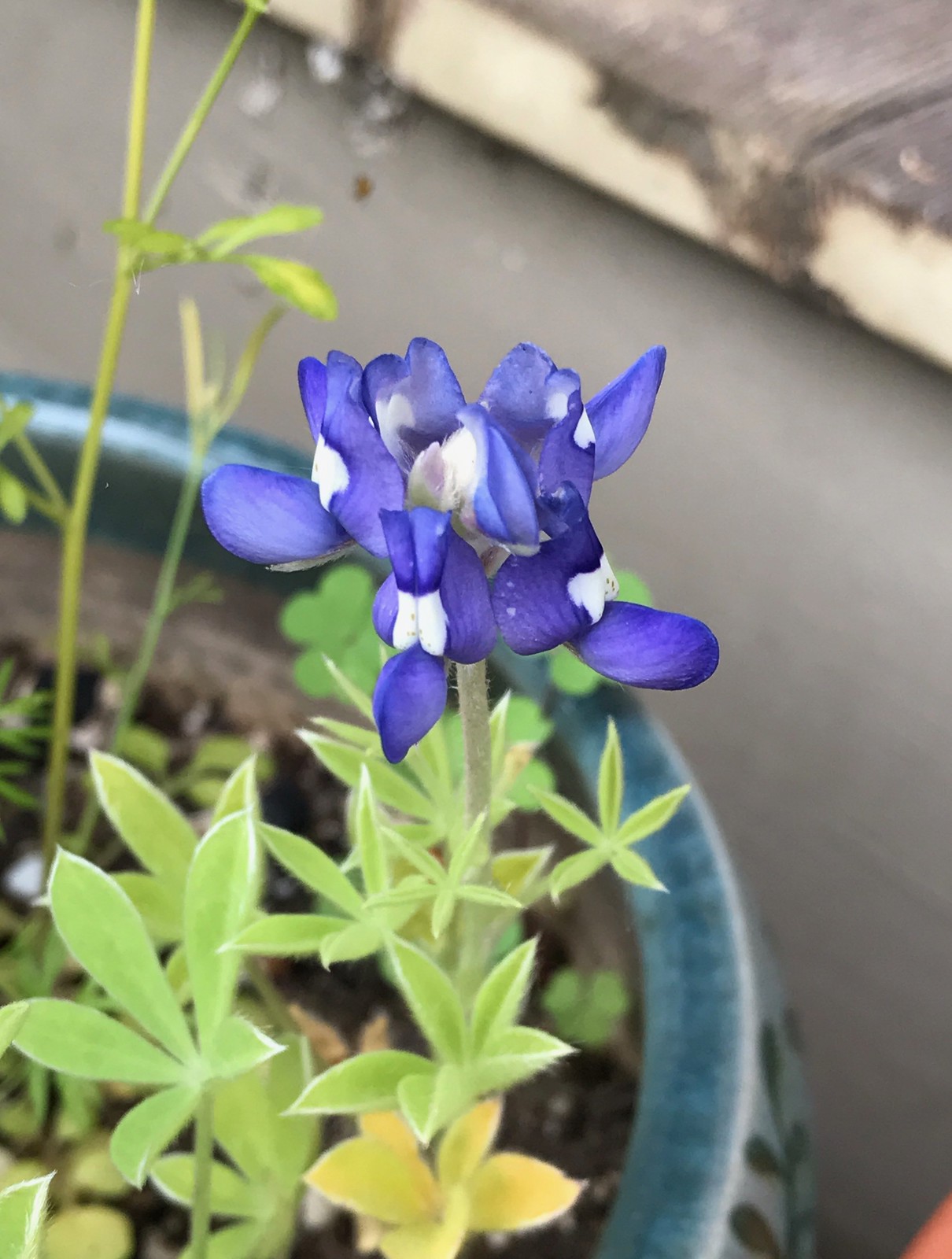The photograph features a vibrant purple-blue flower, consisting of multiple star-shaped blossoms clustered around a green stem. This stem emerges from a dark brown, moist-looking soil contained within a ceramic pot, richly painted in a dark teal hue with a green floral pattern adorning its sides. The pot is placed on a black asphalt surface, suggesting an outdoor setting. In the composition's top right, there's a partially painted brown wooden plank platform and a small orange fragment near the bottom right, adding subtle details to the scene.